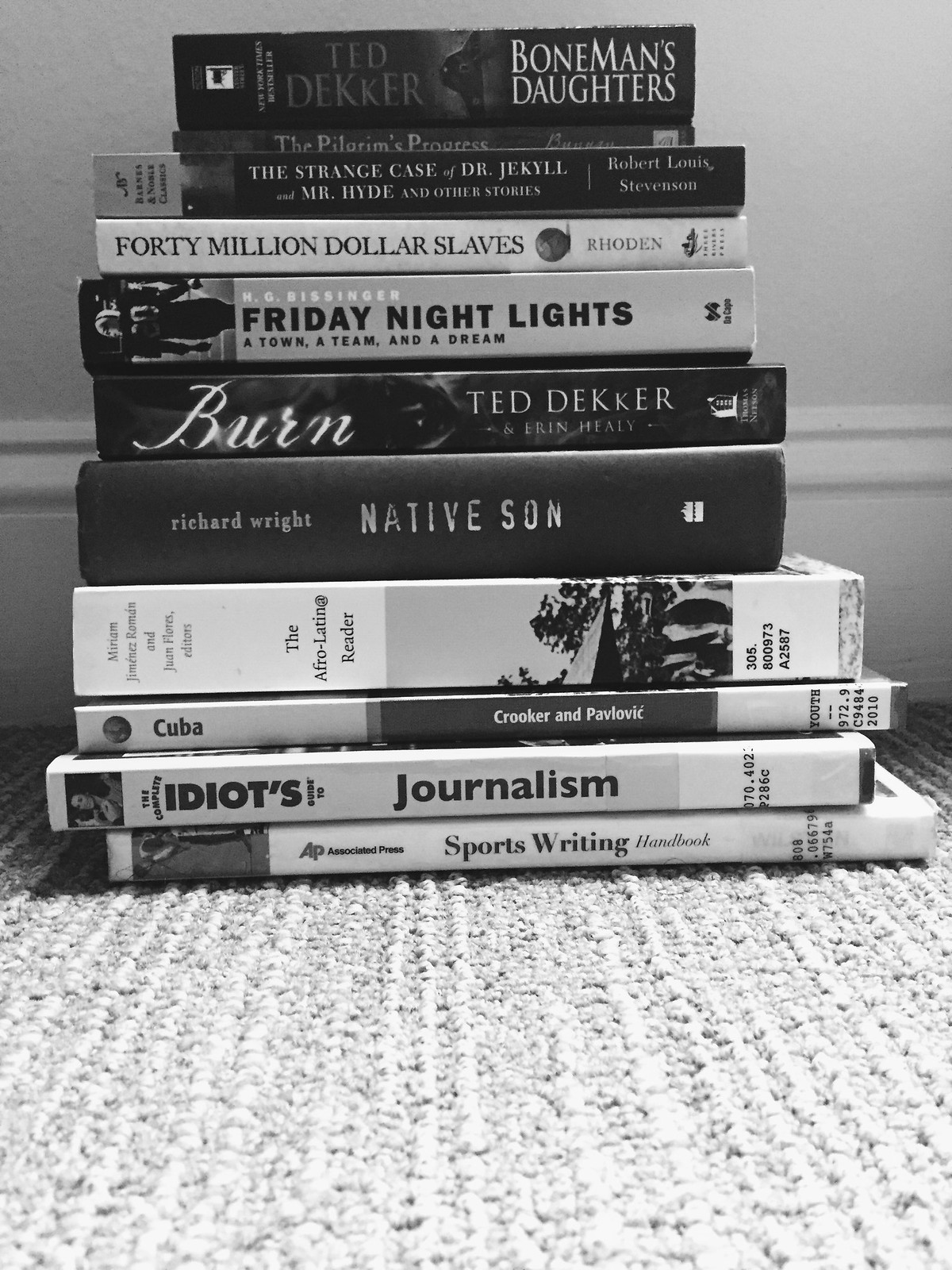This black and white image captures a neatly stacked pile of approximately 11 books resting on a carpeted floor. The stack is positioned centrally in the image, against a backdrop of a white baseboard and a slightly darker hued wall—though the black and white palette makes the exact colors indeterminable. The books vary in size, starting smaller at the top and increasing in size toward the bottom. The visible titles and authors from top to bottom include: "Bone Man's Daughters" by Ted Decker, "The Strange Case of Dr. Jekyll and Mr. Hyde", "40 Million Dollar Slaves", "Friday Night Lights", "Native Son", "The Afro-Latin Reader", "Journalism and Sports Writing". The detailed text on the sides of the books adds a scholarly touch to the composition, which appears to be an indoor setting with no additional objects present.